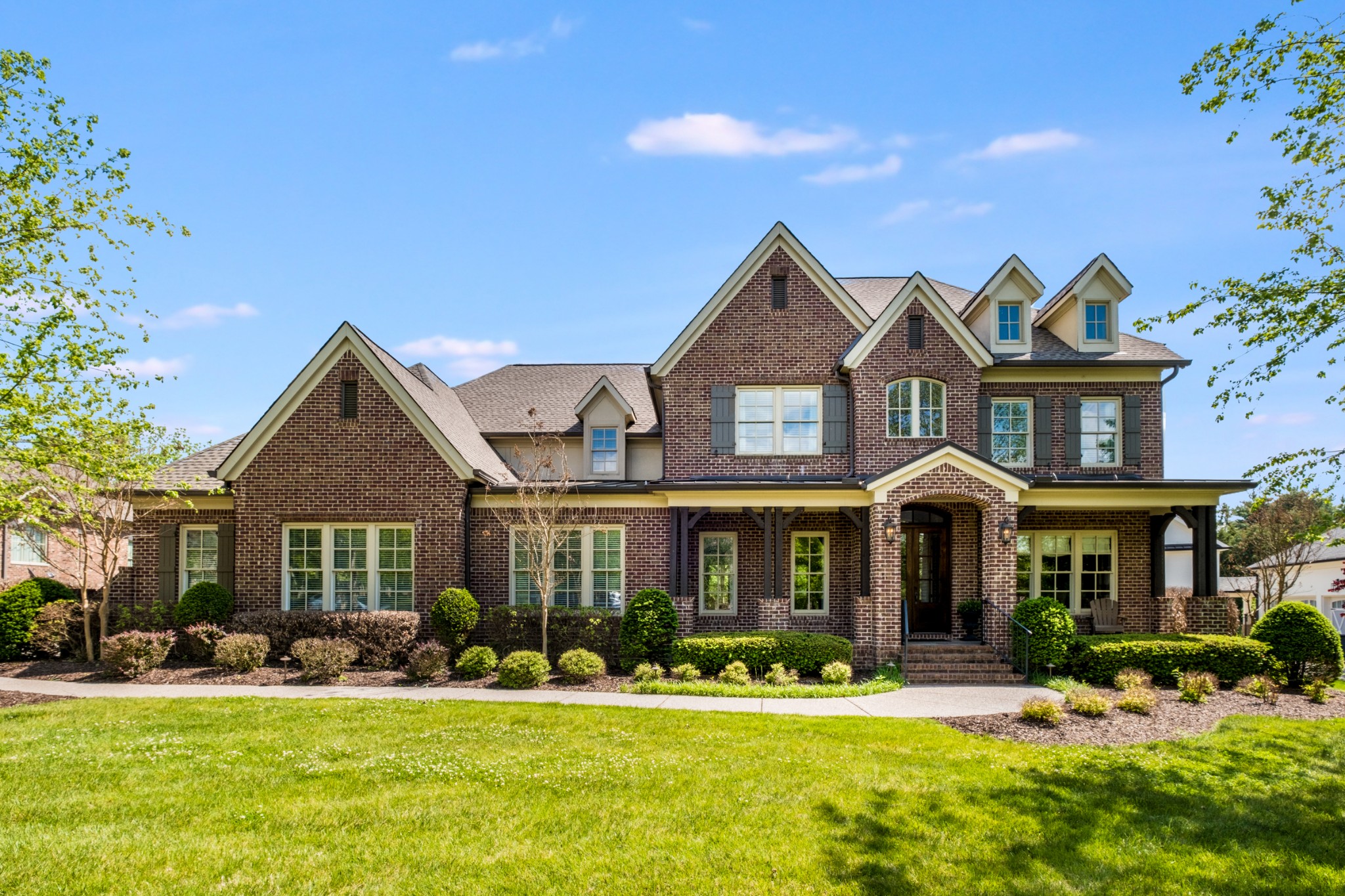The image depicts an elegant, large two-story brick house under a clear blue sky with a few white clouds. The front lawn, with its bright and freshly colored green grass, occupies the lower quarter of the picture, while the house itself dominates the central portion. The house features numerous triangular-shaped roofs, with a total of five distinct peaks adding to its architectural charm. An arched entryway, set back, leads to a grand porch supported by pillars. French windows adorn the façade, with about a dozen on the ground floor and approximately five on the upper floor, suggesting a well-lit interior. At the very top, small windows hint at an attic space. Surrounding the house, neatly trimmed bushes and shrubbery enhance its curb appeal. Two barely visible trees flank the sides, and a small tree stands in front, near a curved paved walkway that leads to the porch. On the right side, there appears to be a patio area, contributing to the house’s overall luxurious feel.